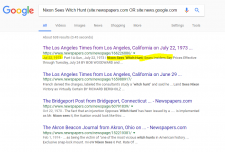This image displays a screenshot of Google search results, characterized by the iconic multicolored Google logo located in the upper left corner. The logo features a light blue 'G', a red 'o', a yellow 'o', a blue 'g', a green 'l', and a red 'e'. Directly below the logo is the elongated search bar, filled end-to-end with a lengthy query. Adjacent to the search bar are icons for a microphone and a magnifying glass, the latter symbolizing the search function. Beneath the search bar is the Google menu, highlighted by various tabs such as "All," "Video," and "Images," with the "All" tab being prominently active. The search results are segmented into four distinct sections, each reflecting different links and information related to the query. Due to the reduced size of the image, the text and finer details are challenging to discern.